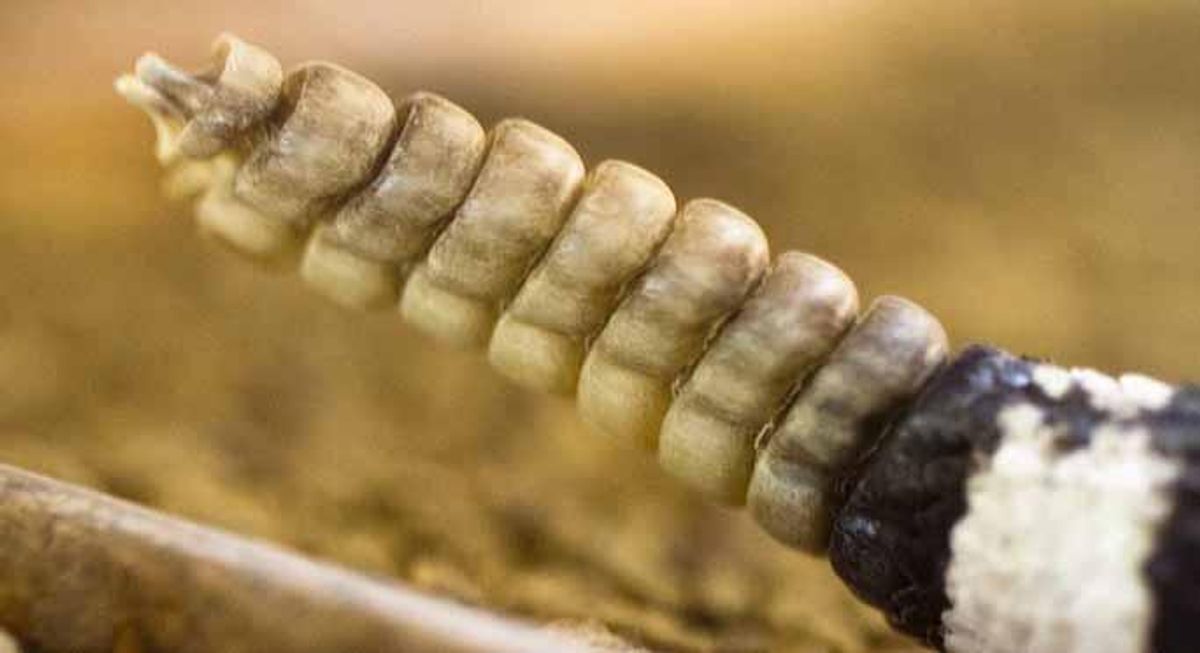This extreme close-up macro photograph captures the segmented rattler of a rattlesnake, prominently displayed against a blurred, light tan background. The rattler, comprised of a series of interlocking circular segments, appears to be made of organic material possibly resembling bone, with a light olive green coloration and distinct blackish lines. These segments are slightly twisted at the top, with two pieces pointing straight out. Emerging from the bottom right-hand corner, the rattlesnake's scaly tail features striking black and white scales, highlighted by a thick white line marking the transition to the rattler. The blurred backdrop adds a swirl of amber and brown hues, suggesting a natural ground covering, yet keeping the rattlesnake's menacing tail as the clear focus.